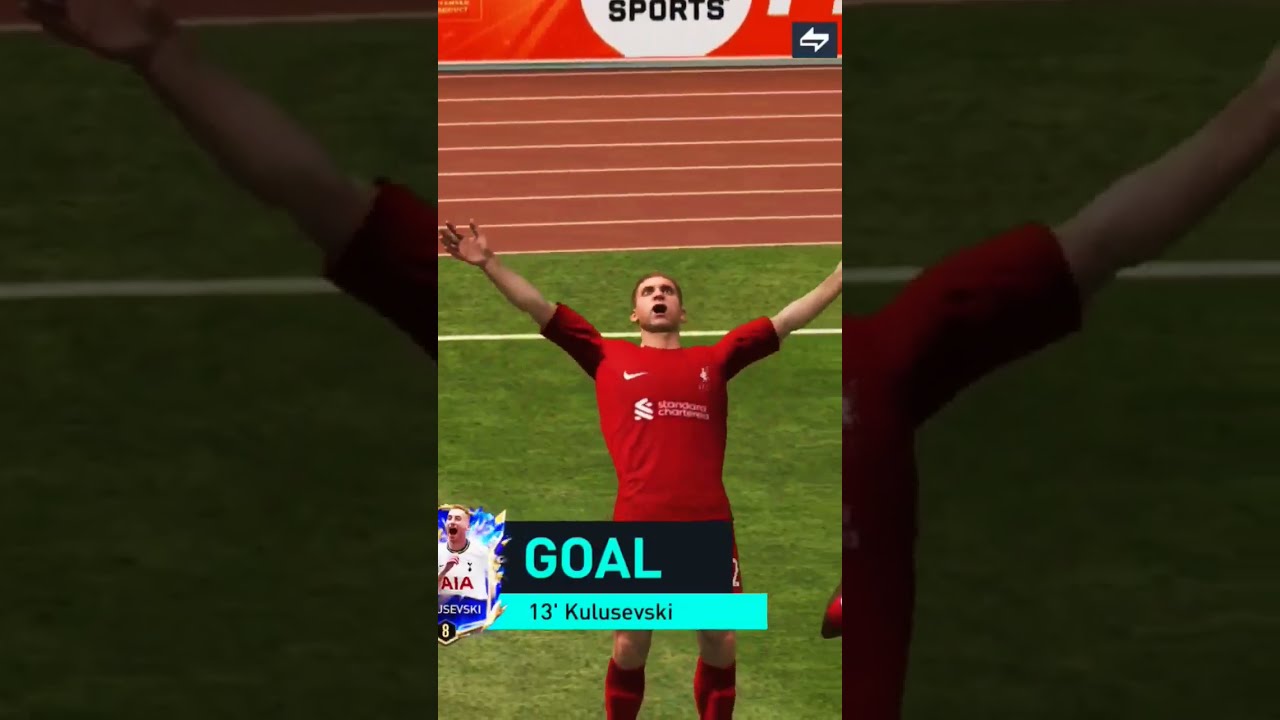This is a detailed screenshot of a soccer video game, possibly FIFA, which appears to be captured on a smartphone and spliced into three distinct, smartphone-sized rectangles. The central rectangle is fully colored, while the side rectangles are grayed out. The focal point of the image is a soccer player, Dejan Kulusevski, animated in a victorious pose with his arms raised towards the sky as if celebrating or cheering. He is wearing a red Nike shirt with additional designs beneath the brand logo. The scene is layered with a dark filter, with the central image brightened. At the top of the image, within a white circle flanked by orange, is the word "sports." The bottom left corner features a small bar reading "Goal 13 (Kulusevski)," alongside a unique player card. The scene depicts a moment of triumph on the green soccer field, adding a dynamic and spirited vibe to the image.